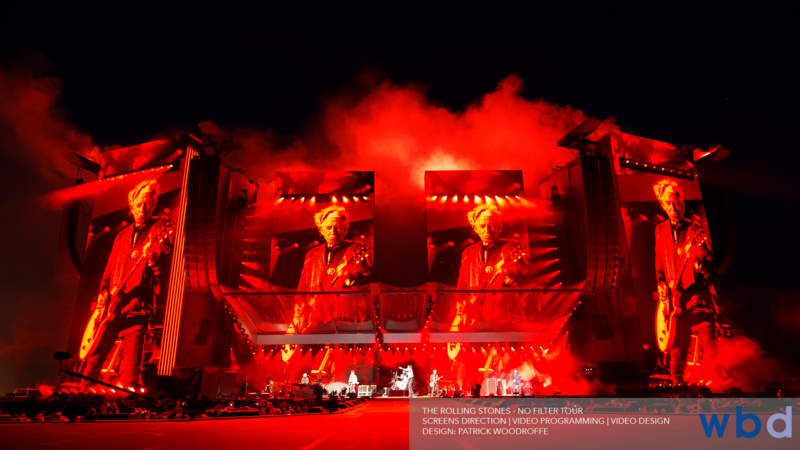The advertisement showcases the Rolling Stones' No Filter Tour. Dominated by vibrant red tones with accents of bright orange and yellow flames, the image has a dynamic and electrifying atmosphere that exudes heat and excitement. Four massive screens display larger-than-life images, likely of Keith Richards, each capturing different angles but maintaining the same pose, suggesting a live performance aura. Beneath the two central screens, the band plays, surrounded by pyrotechnics that fill the scene with an intense glow.

The background is predominantly black, adding to the dramatic contrast of colors and heightening the overall impact. The audience is visible, positioned at an eye-level with the catwalk, which extends into the crowd, suggesting an intimate and immersive concert experience possibly set in a large stadium.

At the bottom of the image, white text on a red background lists the details: "The Rolling Stones No Filter Tour, Screens Direction, Video Programming, Video Design. Designed by Patrick Woodroffe." Additionally, the initials WBD appear in lighter blue, providing a hint of the production and creative teams behind the visuals. This elaborate setup not only advertises the tour but also highlights the meticulous design and video elements curated by Patrick Woodroffe, capturing the grandeur and intensity of a Rolling Stones live performance.